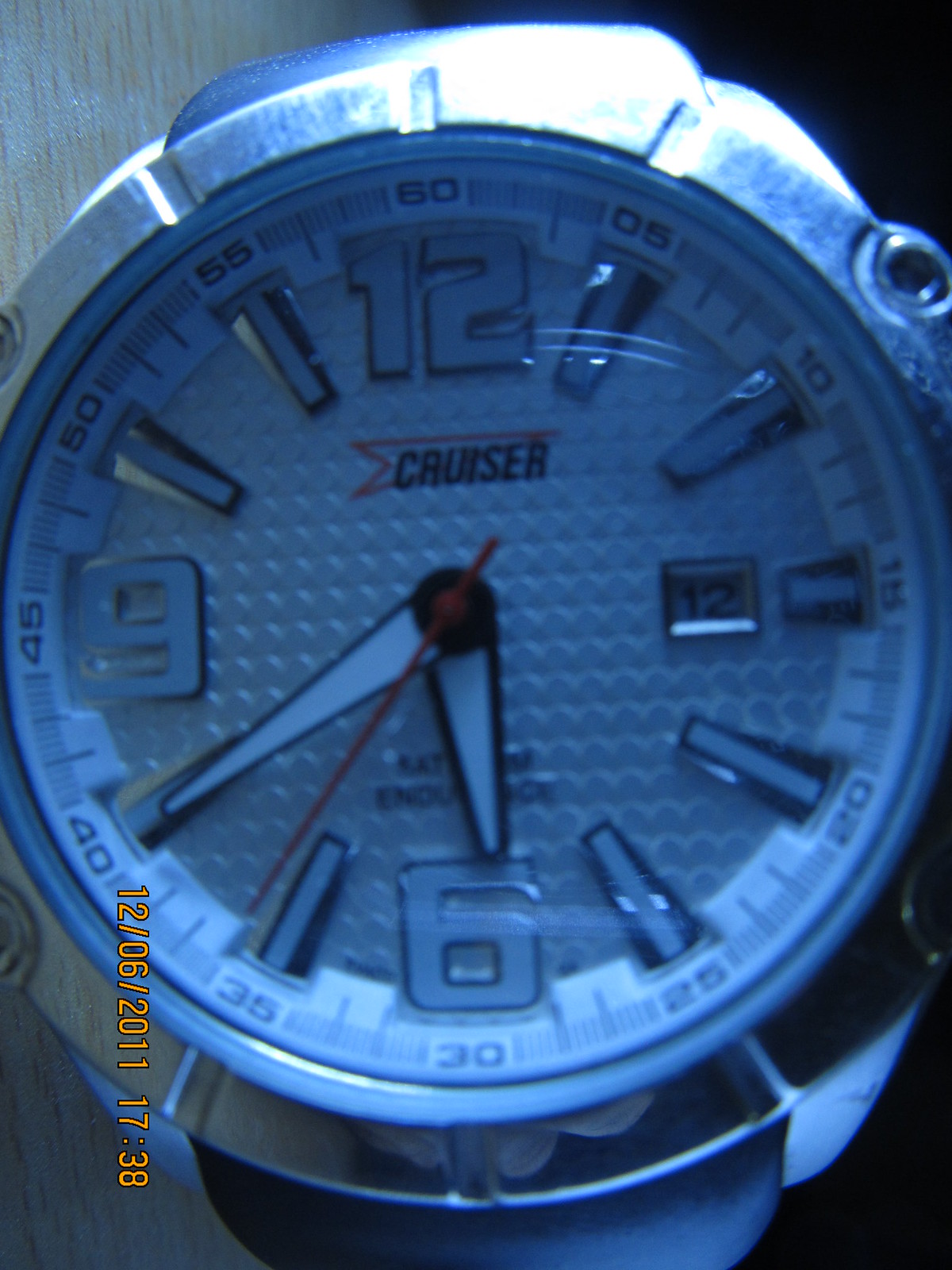Close-up Image of a Well-Worn Diver's Watch: 

This photograph, captured on December 6, 2011, at 17:38, features an up-close view of a silver diver's watch, displaying its detailed craftsmanship and signs of use. The watch is encased in a robust silver frame with distinctive indentations encircling its perimeter. The dial suggests functionality pertinent to a diver's watch, allowing the user to rotate and align various numbers. The watch face is white, adorned with numerals outlined in silver, enhancing readability. The watch hands are primarily white with black outlines, ensuring clear visibility against the white backdrop. The red second hand adds a striking contrast and precision to this timepiece. 

Central to the face is the brand name "C-A-U-I-S-E-R" rendered in black text, accompanied by a prominent red insignia, signifying its unique make. Evident wear and tear, manifested as numerous scratches, authenticate the watch's use over time. Additionally, the image includes a visible reflection, likely caused by a light source, further enriching the texture and realism of the photograph.